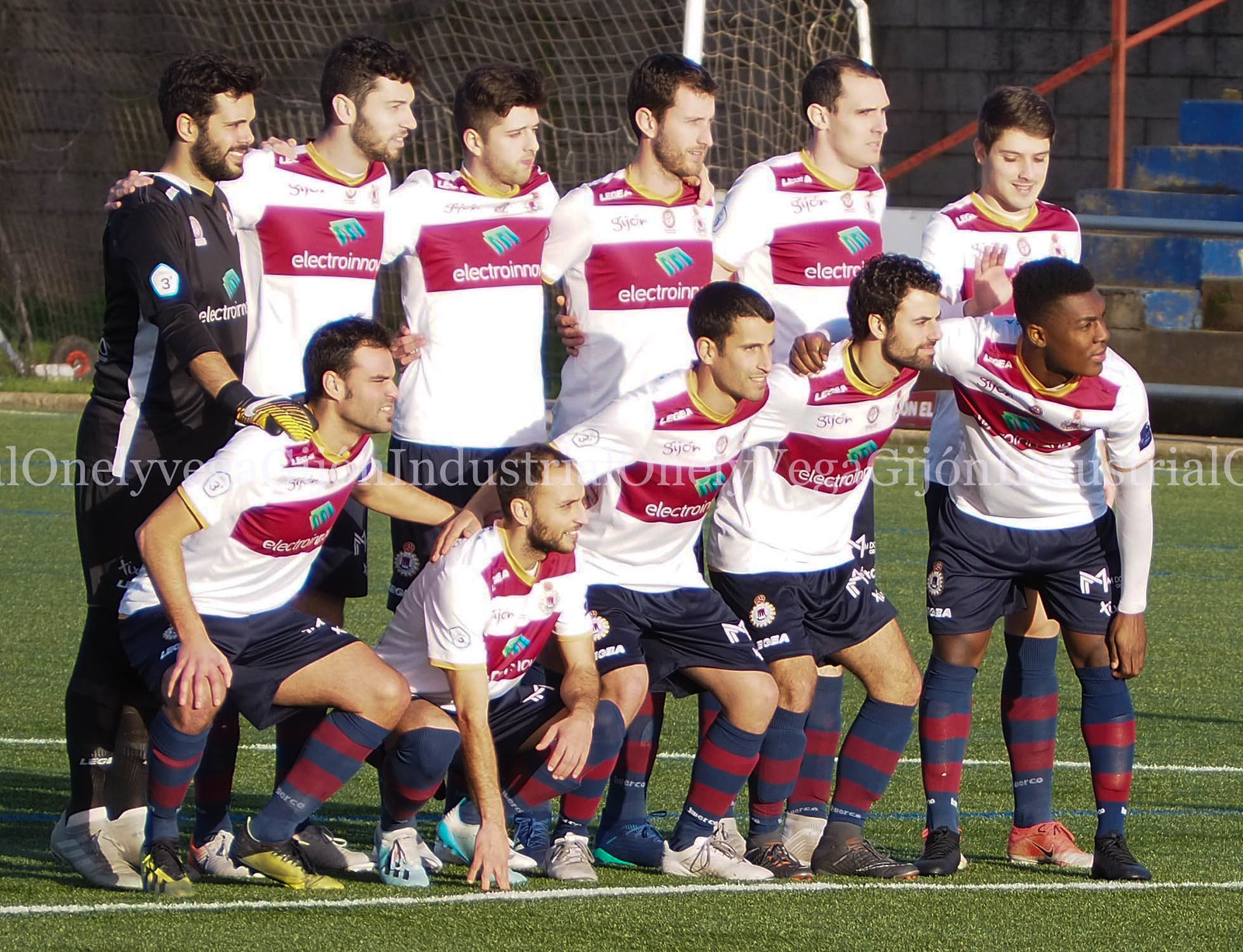This is a horizontal rectangular image of a soccer team posing for a photograph on a green grass field. The team comprises several young men wearing white t-shirts with a red emblem across the front that says "Electronica," paired with navy blue shorts and tall red and blue striped socks. Most players wear white shoes, though some sport different colored footwear. They are organized in two rows: the front row is kneeling, with some players crouched down and touching the ground, while the back row is standing with their arms around one another. Notably, a person in a black uniform stands at the far left, likely the coach or trainer, distinguished by black and yellow gloves. In the background, the photo features a soccer net and blue bleachers with an orange pole, indicating the spectator area. The entire team appears to be looking slightly to the left, collectively posed and ready for action.